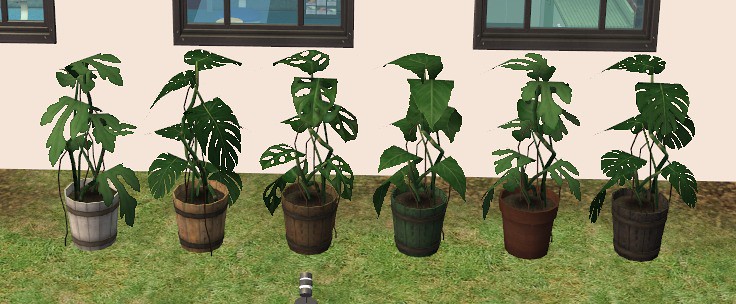The image showcases a computer-generated scene of the exterior of a house-like structure painted yellow. The structure features three windows with black frames, partially cut off at the top of the image, offering no clear view inside. In front of the structure lies a neatly manicured, albeit artificial-looking, grassy lawn with some dirt patches. Six flowerpots of varying colors—including shades of gray, green, and brown—are evenly spaced along the lawn. Each flowerpot contains a healthy green plant with large leaves. Notably, there is an indistinguishable white and silver object positioned in front of the third plant from the left. The entire scene gives off a noticeably digital, pixelated quality, indicative of it being a screenshot from a computer program rather than a photograph or hand-drawn/painted image.